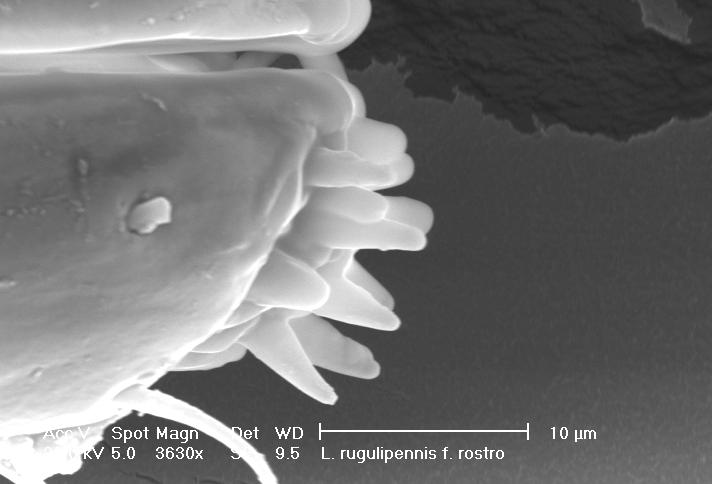The image is a highly magnified, microscopic view of a white and gray underwater organism with tentacle-like protrusions extending from the left side towards the center. The organism appears as a large, rounded blob with multiple carrot-shaped extensions. The background is predominantly black, with a prominent black splotch in the upper right corner that resembles an island when viewed from above. At the bottom of the image, there is white text displaying statistical data about the photograph. The text includes information such as "ACOV spot MAG-N," "33630 times magnification," and "10 µm," along with other words and numbers indicating specifics related to the magnification and possibly the photographer's name, like "Rugu L. Penis F. Rostro." The overall aesthetic is a stark contrast between the white and gray organism and the dark background, with detailed textual information enhancing the scientific context.